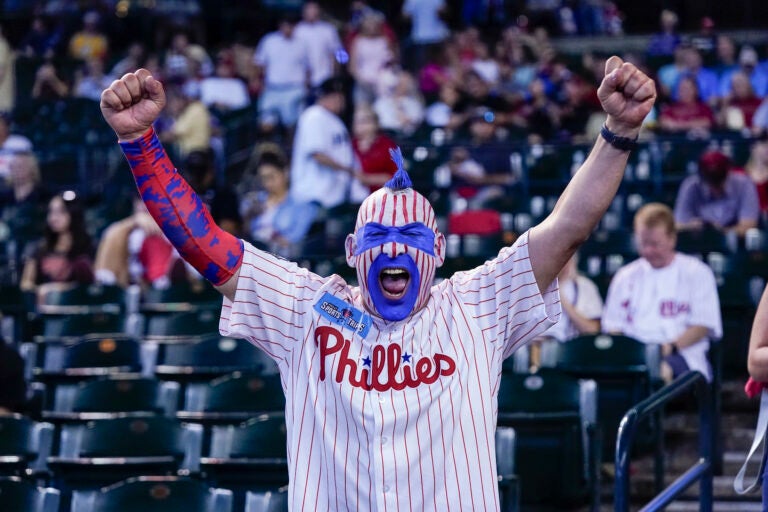The image captures a fervent Philadelphia Phillies fan in the stands, animatedly cheering with both fists raised high. He is dressed head-to-toe in Phillies gear, prominently featuring a white Phillies jersey with red stripes and "Phillies" written in red cursive text, accentuated by two stars. His face is elaborately painted to match his jersey, with white as the base color, red stripes, and blue accents around his eyes and mouth, creating a mask-like effect. Complementing his enthusiastic look, he wears a red and blue spandex sleeve on his right arm and a black watch on his bare left wrist. His purple hair adds to his vivid appearance. The background reveals a blurred crowd of calm and seated fans, further emphasizing the energetic demeanor of this standout supporter.